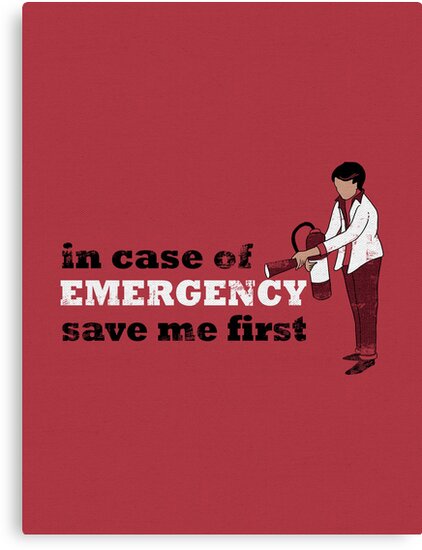The image is a computer-generated illustration featuring a vintage sign with weathered text displayed against a rich red background. On the left side, the sign reads "in case of" in black letters, followed by "EMERGENCY" in large white capital letters, and "save me first" again in black letters. The text is organized in three lines, adding to an aged look. On the right side of the image stands a faceless, illustrated woman with a short, tapered brown haircut. She wears a light cream-colored jacket over a dark red burgundy shirt and pants, completed with black shoes. The woman holds a red fire extinguisher with a white label, directing the nozzle towards the word "EMERGENCY." The overall artwork appears as though it could be a humorous or ironic sticker or wall sign.